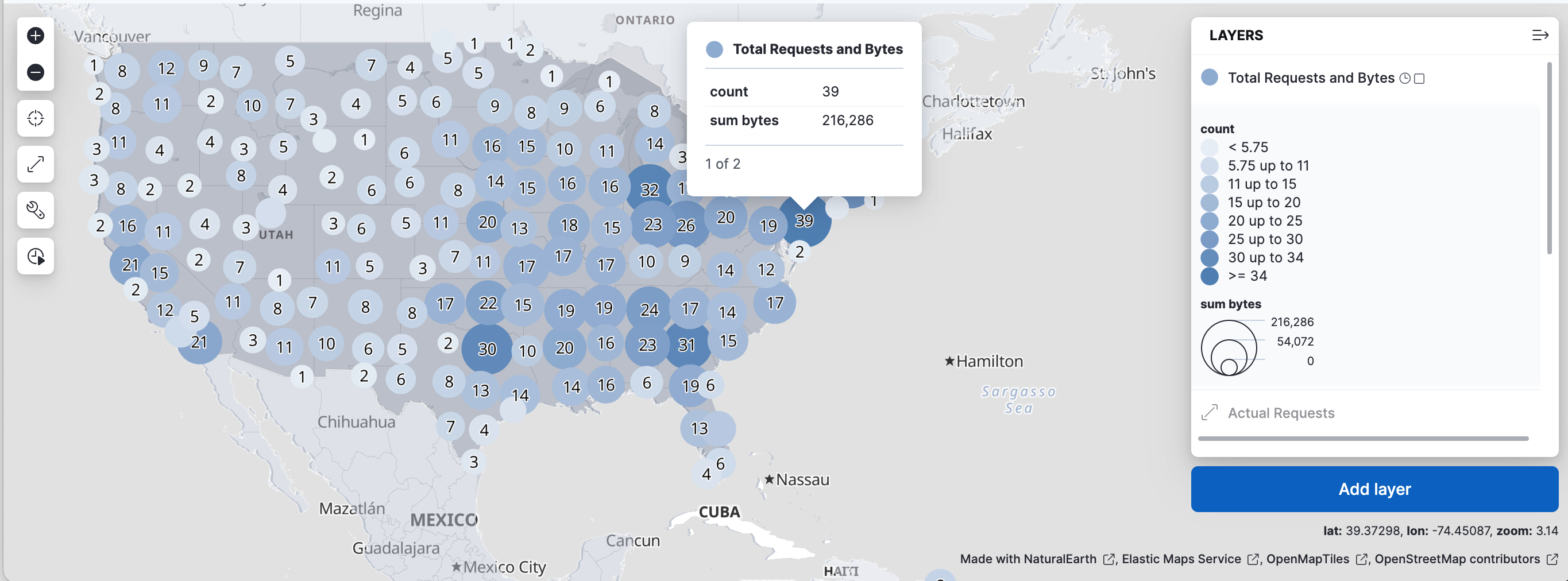This image is a detailed screenshot of a map of the United States, overlaid with various data points, coordinates, and numerical values. The map features different states, each marked with specific data. On the right side of the image, there are several informational layers. These layers display data segmented into ranges: 5.75 up to 11, 11 up to 15, 15 up to 20, 20 up to 25, 25 up to 30, and 30 up to 34. 

Additionally, the numeric values for bytes are prominently displayed. One notable figure is 216,286 bytes, while the median bytes are shown as 54,072. There's also an interface for adding new layers based on requests and bytes. Centrally located within the screenshot is a summary section presenting total requests and bytes, highlighting a count of 39 requests and a total byte count of 216,286.

Towards the bottom of the screen, the pagination indicator shows '1 of 2,' suggesting multiple pages of data. Overall, the entire screenshot is formatted in a long rectangular layout, capturing all the described elements in detail.